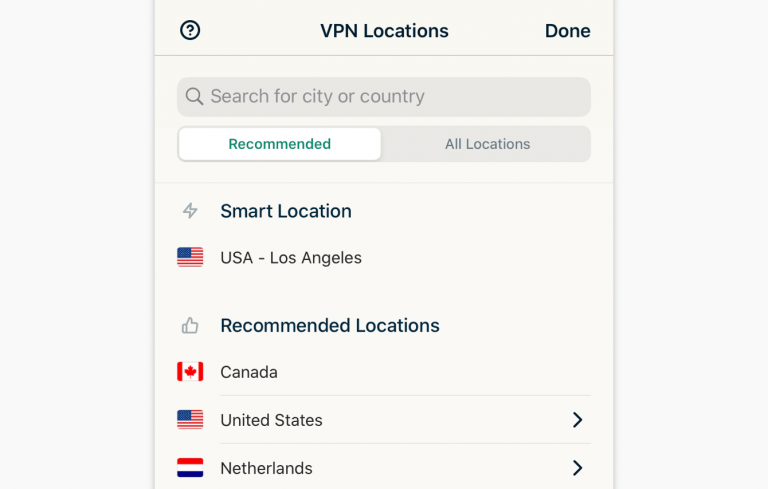In the upper left corner of the display, there is a question mark icon enclosed within a circle, indicative of a help or informational feature. Adjacent to this icon, the text "VPN LOCATIONS" is prominently displayed in all capital letters. Towards the upper right corner, the word "Done" is positioned. 

Below this section, within a gray search bar, the placeholder text "Search for City or Country" is visible. Following this is a white box containing the word "Recommended" in green text, while to its right, in a lighter gray shade that indicates it is not currently active, it says "All Locations."

Moving downwards, the black text "Smart Location" is visible. Underneath this, there is an illustrative image of the American flag, showcasing its stars, stripes, and traditional red, white, and blue colors. To the right of the flag, in all capital letters, it reads "USA - Los Angeles." Below this entry, there is a small gray thumbs-up icon, signifying a recommended choice. Directly to the right, the label "Recommended Locations" is given.

Next, the flag of Canada appears, characterized by a red maple leaf and red and white stripes. Beside this flag, the word "Canada" is shown. Below, another representation of the United States flag is displayed with the text "United States" adjacent to it.

Finally, a flag with horizontal red, white, and navy blue stripes, representing the Netherlands, appears in a square. Beside the flag, the word "Netherlands" is noted. To the right of these listings, an option to click a right arrow is present, likely for expanding the list or navigating further.